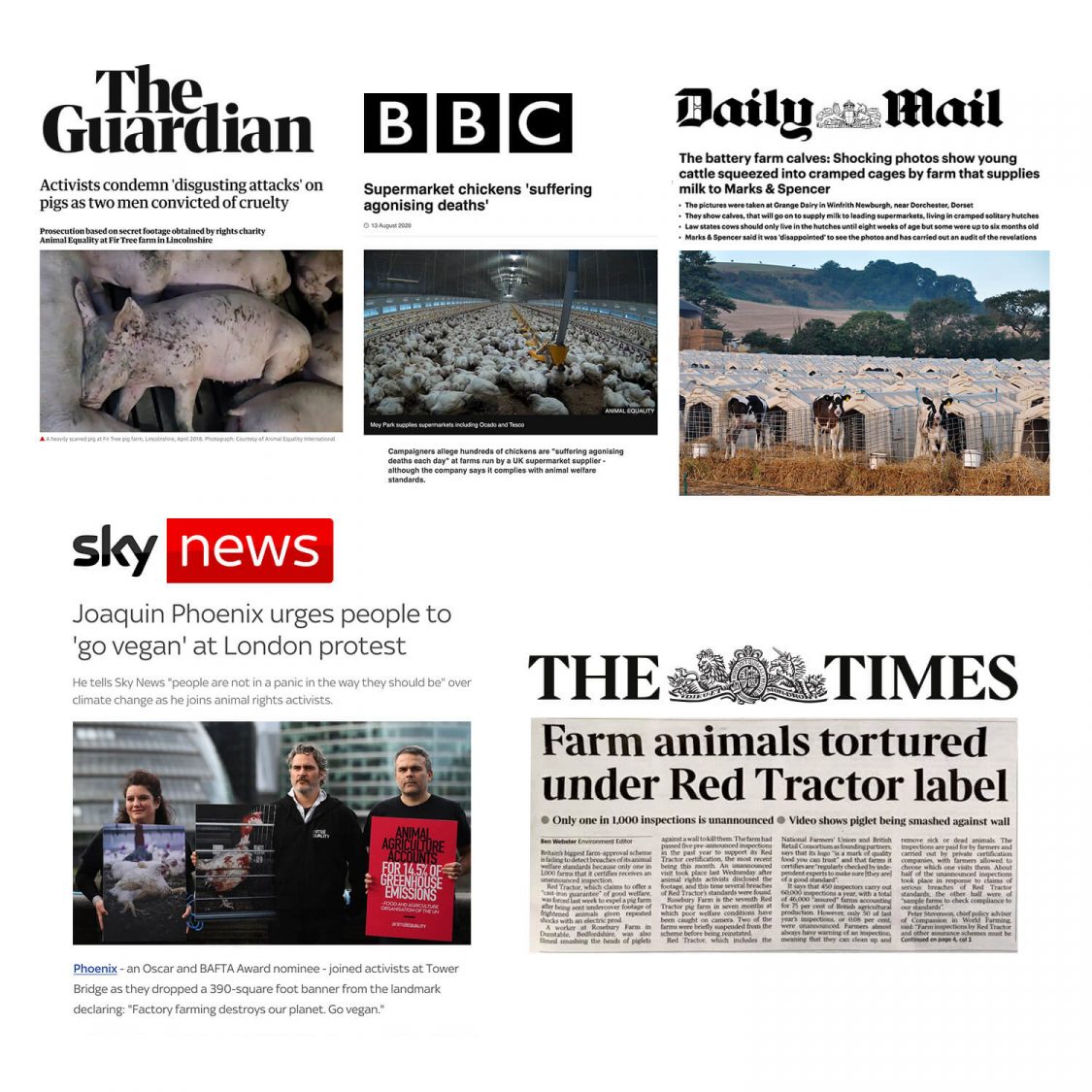A collage of various news articles highlights the widespread attention to animal cruelty across different media outlets. The top of the image features a screenshot from The Guardian, presenting a headline: "Activists condemn 'disgusting' attacks on pigs as two men convicted of cruelty," accompanied by a heart-wrenching photo of an injured pig. To the left, a BBC article titled "Supermarket chickens suffering agonizing deaths" is shown, with a distressing image of an overcrowded indoor space filled with white chickens. On the right, a Daily Mail article showcases the headline "The Battery Farm calves: Shocking photos show young cattle squeezed into cramped cages by farm that supplies milk to Marks and Spencer," featuring a poignant picture of calves looking directly at the camera from their cramped enclosures. 

At the bottom of the collage, Sky News captures attention with its bold red and white text: "Joaquin Phoenix urges people to go vegan at London protests," accompanied by a photo of actor Joaquin Phoenix with two other individuals at the protest. Finally, on the bottom right, The Times displays a grave headline on a gray background: "Farm animals tortured under Red Tractor label," bringing to light the harsh conditions under a supposed quality assurance scheme.

The amalgamation of these headlines underscores a collective outcry against the mistreatment of farm animals, portraying a grim reality that animal rights activists around the world are striving to change.